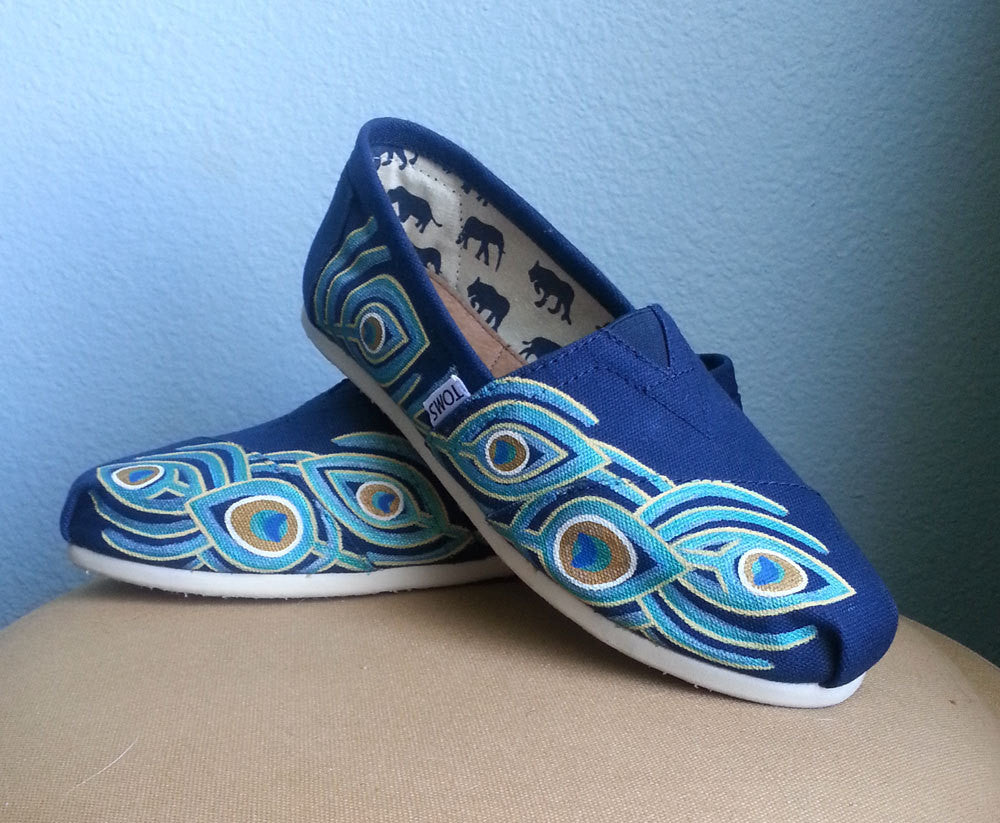This image captures a pair of TOMS canvas shoes, showcasing a handmade aesthetic while carrying a designer's touch. The shoes are primarily dark blue with a distinctive light blue peacock feather design that cascades down the sides. These designs resemble teardrop shapes adorned with concentric circle lines, giving a whimsical and artful appearance. A white label on the side of the right shoe reads "TOMS," enhancing the brand's identity. The shoes' inner linings are white, featuring intricate dark blue animal prints, including elephants. The shoes rest on a tan fabric-covered platform or cushion, with the right shoe's heel gently resting on the left shoe, all set against a serene light blue wall. The soles of the shoes are white, completing the elegant yet casual look.